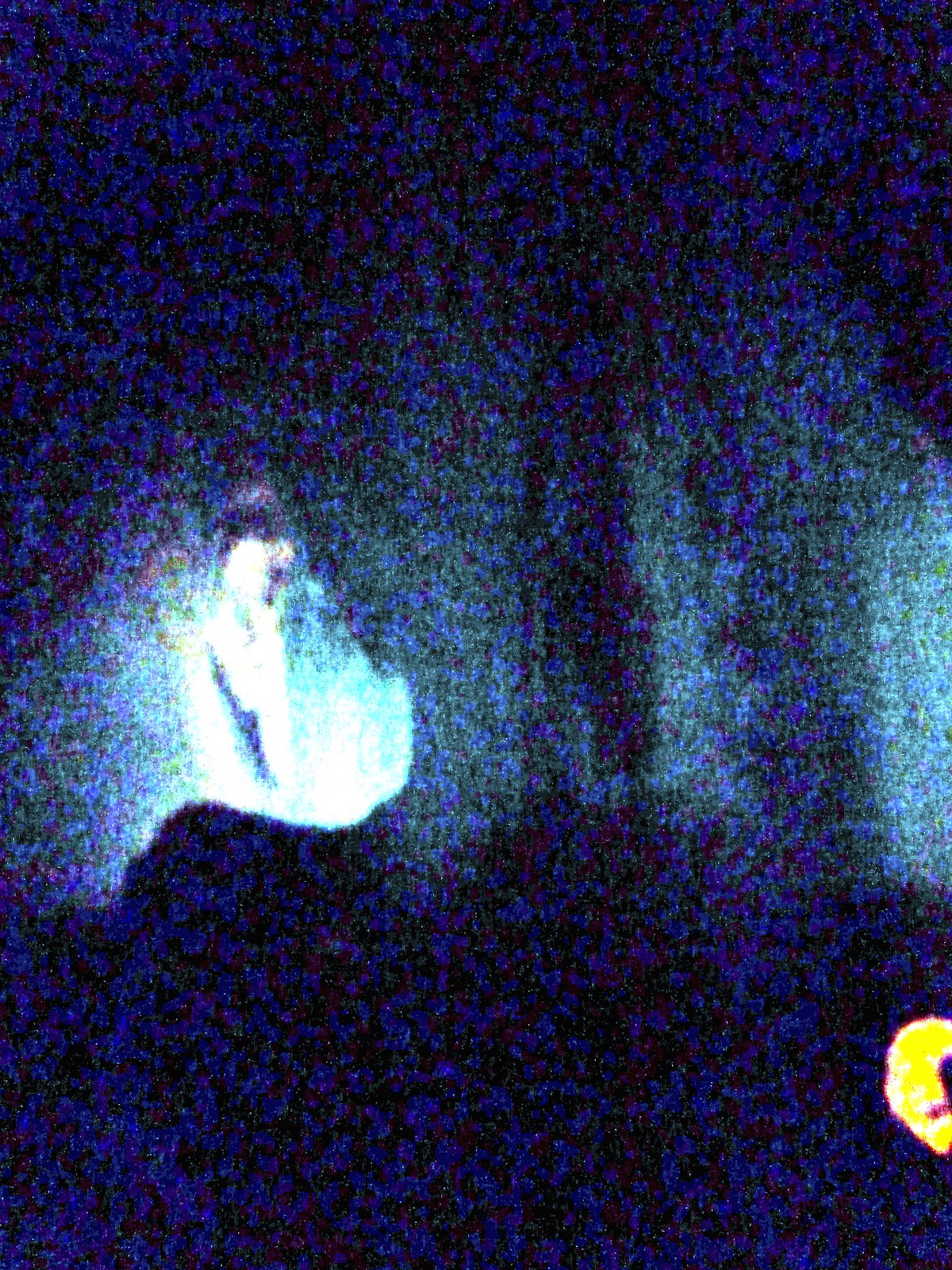This is a vertical, rectangular painting with a predominantly black background, executed in a pixelated style. The composition is primarily made up of royal blue pixels, which appear sparser at the top and gradually become denser as they descend to the midpoint of the painting. Interspersed among these blue pixels are white pixels, which, on the left side of the middle section, cluster so densely that they resemble a passageway. This area of concentrated white pixels subtly transitions into a soft tealy blue color in the background, adding a calming nuance to the piece.

Across the middle section, additional white pixels create a scattered yet noticeable pattern, with a particularly dense collection on the right side, maintaining the overall pixelated aesthetic. At the very bottom, the royal blue pixels are packed tightly together, forming almost blob-like images. Notably, in the bottom-right corner, a crescent-shaped collection of yellow pixels emerges, peeking onto the edge of the canvas and adding a striking contrast to the surrounding blues and whites.